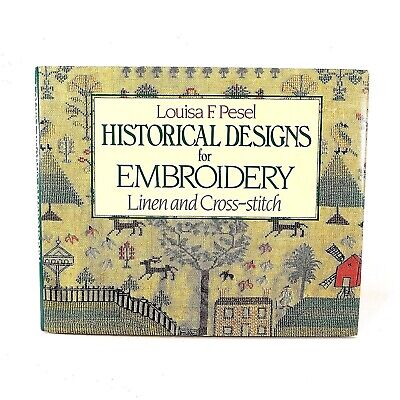The cover of the book, which is aimed at teaching embroidery, is primarily a pale yellow color adorned with intricate embroidered designs. These designs feature an idyllic landscape comprising a variety of elements: a house positioned at the bottom, flanked by trees, a hill with a gate to the left, and a windmill perched on another hill to the right. The scene is dotted with pixelated pine trees and running deer, contributing to an overall pattern rather than a narrative. A prominent black border in the center encloses a white square with dark blue font, where the title reads, "Louisa F. Purcell, Historical Designs for Embroidery, Linen and Cross Stitch." Additionally, the bottom right corner of the cover features a red birdhouse, enhancing the rural theme of the illustration.